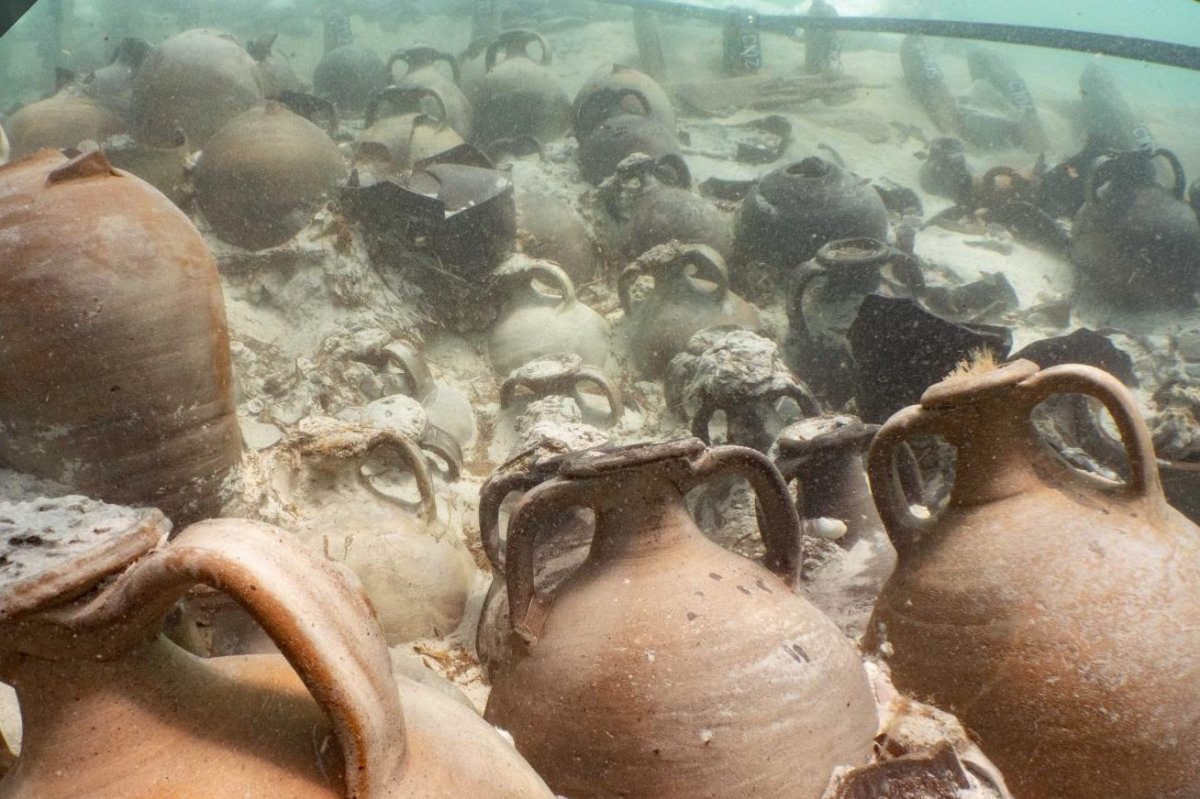This underwater photograph showcases a remarkable scene of ancient Roman ceramic wine jugs, beautifully preserved, nestled within the remnants of a centuries-old shipwreck. The jugs, each with two handles and a narrow neck, exhibit a range of colors from dark brown to reddish-brown, with some partially submerged in sand and silt. The foreground features four prominently visible jugs, while dozens more can be seen scattered in the background, some intact and others broken. The underwater environment is rendered in stunning detail with ribs of the ship faintly visible amid the sand, and the water appears cloudy with white and brown specks drifting through the scene. This image captures a moment of ongoing recovery efforts as divers carefully excavate these 1700 to 2000-year-old artifacts, offering a glimpse into the rich history of ancient maritime trade.